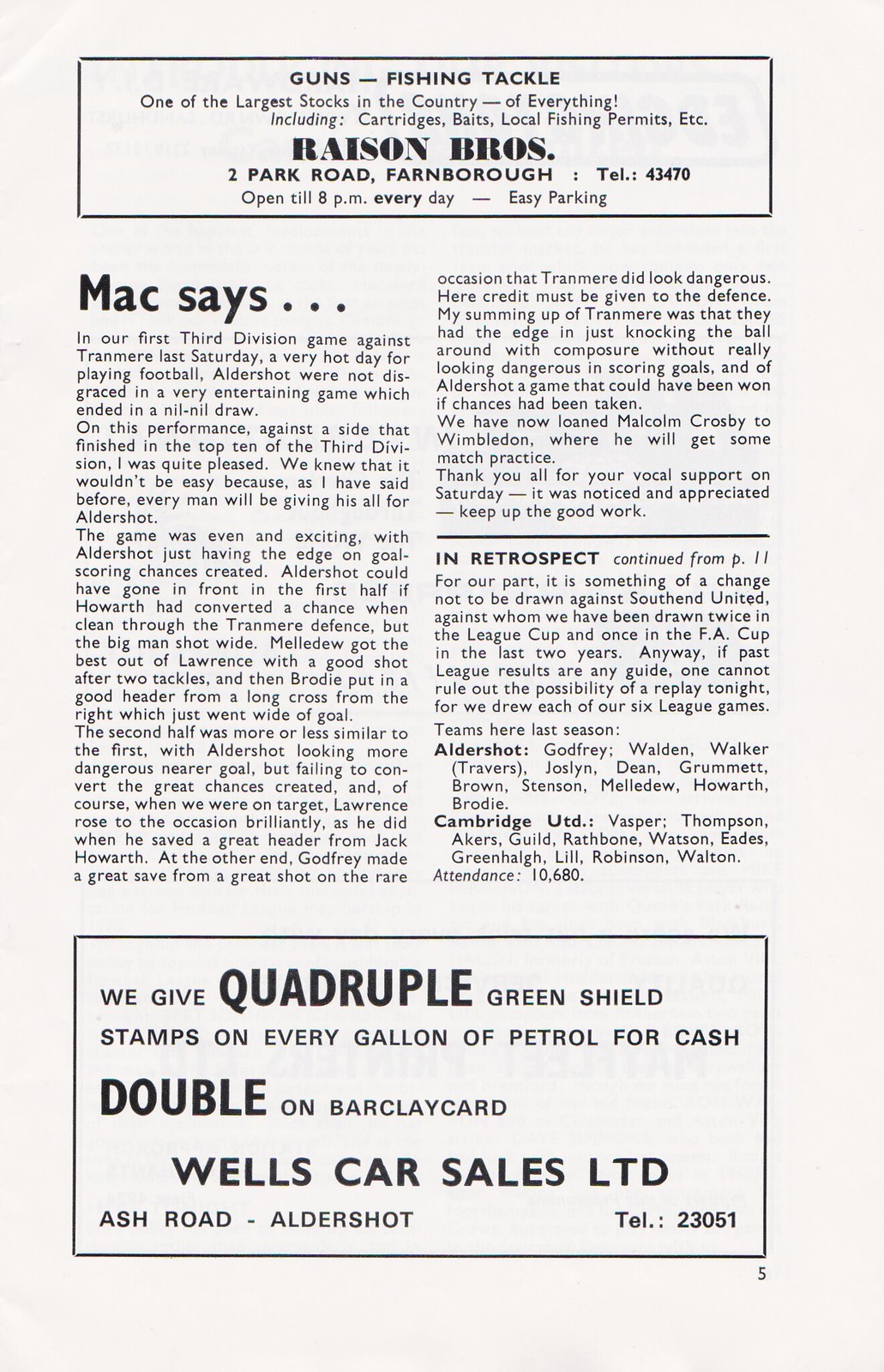This image, sourced from a magazine, prominently features a detailed advertisement at the top of the page for Raisin Brothers, located on Tupac Road, Farnborough. The ad highlights their extensive inventory of guns, fishing tackle, cartridges, baits, and local fishing permits, positioning them as having one of the largest stocks in the country. The store offers easy parking and remains open until 8 PM daily, with a contact telephone number of 43470.

Beneath this advertisement, the page contains an article section titled "Max Says," presented in two columns. At the bottom of the page, there is another advertisement from Wells Car Sales Limited, located on Ash Road, Aldershot. This ad promotes their offer of quadruple Green Shield stamps on every gallon of petrol for cash transactions, and double stamps for Barclay Card purchases, with a contact telephone number of 23051."